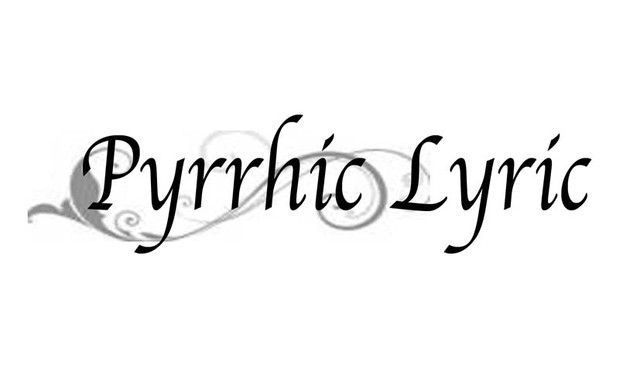Set against a pristine white background, this horizontal, borderless image prominently features the elegant text "Pyrrhic Lyric" in an exquisite black script with the first letters capitalized. The font exudes a refined and fancy aesthetic. Beneath the word "Pyrrhic," there is a sophisticated decorative element rendered in gray – a swirling pattern resembling a flower, stem, or vine, which starts small on the left and progressively enlarges towards the letters "L" and "C" of "Lyric." This delicate gray embellishment provides an artistic touch, complementing the text above it. The overall composition gives the impression of a sophisticated album cover or promotional poster for a musical group, evoking a sense of artistry and grace.